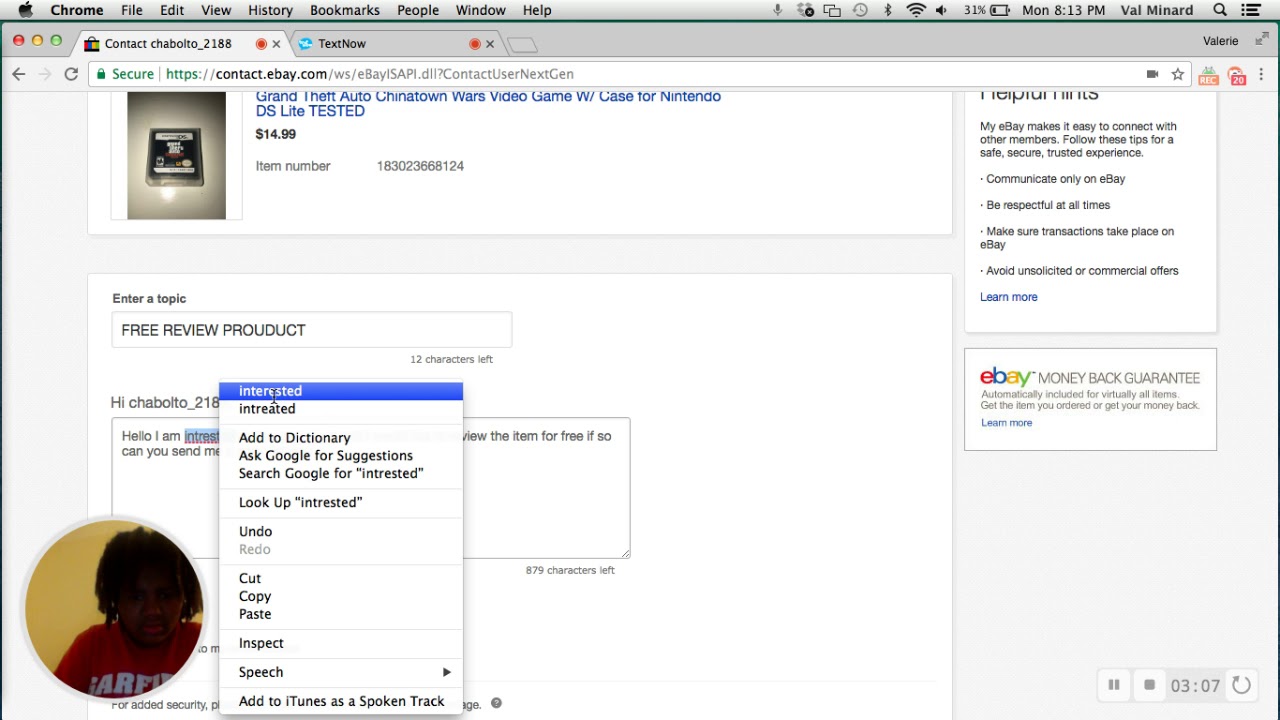This screen-captured image from a website depicts a user interaction on a secure HTTPS webpage, specifically contact.ebay.com. At the center of the interaction is a product inquiry regarding a Grand Theft Auto: Chinatown Wars video game for the Nintendo DS Lite, which includes the game's case and has been tested for functionality. The item is listed for $14.99.

As the user scrolls down, they have selected a topic titled "Free Review Product" and begun typing a message to another user whose screen name is partially visible as "Chilbalto_218." The displayed message reads, "Hi Chilbalto_218, hello I am interested..." but the continuation of this sentence is obscured. However, it suggests the user is inquiring if they can view the item for free or requesting additional details. A profile image visible at the bottom circle shows a person who appears to be an African-American individual with dark hair, though it is unclear whether they are male or female. Additionally, the word "interested" is highlighted, indicating that the user has interacted with this term, with options like lookup, undo, copy, and paste being potentially accessible within the context menu.